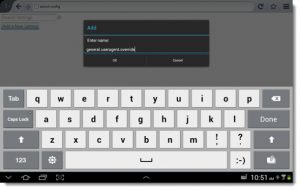A screen capture of a device interface, primarily focusing on a virtual keyboard. The upper portion of the screen showcases an address bar flanked by various icons, including a star, a refresh arrow, and a box. The background appears predominantly white. Overlaying this is a semi-translucent gray pop-up featuring teal and white text. The virtual keyboard covers a significant portion of the image, displaying keys such as "Tab," "Caps Lock," and various others with gray buttons and white text. Additionally, there are keys with gray buttons and black text. The keyboard includes a spacebar, a cogwheel (settings), and functional keys like "X" and "Done." Near the bottom of the image, there's a thin black bar with a series of icons: an arrow, a home button, a stack of papers, a square, and another arrow, with a digital clock showing 10:51 and a battery icon. The image quality is crisp and clear, despite the small size of the screen, with minimal pixelation. The details are sharp, making it easy to identify the elements described.